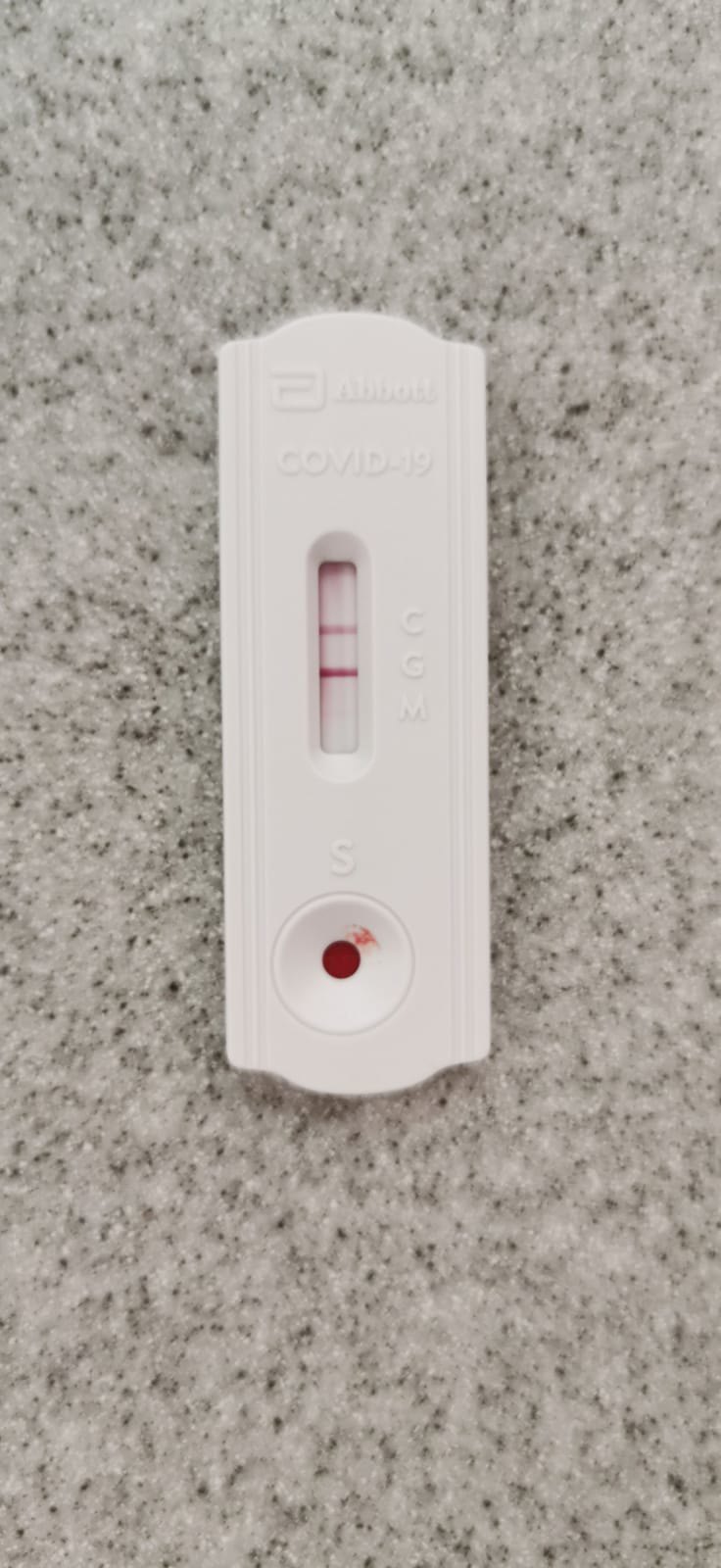This photograph captures a close-up view of a COVID-19 test kit placed on a light gray countertop, which has a pattern of muted black circles and darker gray spots. The centerpiece of the image is the rectangular, white plastic COVID-19 test strip. Both the top and bottom edges of the strip feature low, half-circle ridges rather than a straight, flat edge. 

Near the bottom left of the strip, there is a small, depressed red circle with a slight red smear at the top right of the circle, encased by a white, indented ridge. Just above this circle is a rounded, rectangular depression with a white background. Within this depression, a dark red line runs horizontally across the center, indicating the test result. Above the dark red line, there is a fainter red line also running horizontally, adding detail to the test's reading area. 

The composition and details make it clear that the COVID-19 test strip was used, as indicated by the visible red lines.